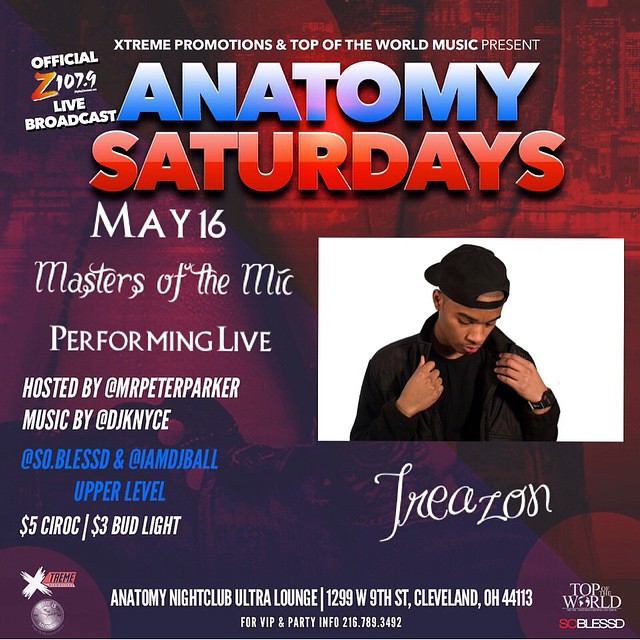Promotional Poster for Anatomy Nightclub Event:

The poster features a vibrant purple and red background with a faded photograph of a city skyline. At the top, in bold white text, it reads "Extreme Promotions and Top of the World Music Present." Directly below, "Anatomy" appears in large blue letters, followed by "Saturdays" in red. In lighter white text, the date, "May 16th," is prominently displayed.

Highlighted beneath the date, in elegant white script, it announces "Masters of the Mic, Performing Live." The event is "Hosted by Mr. Peter Parker" with "Music by DJ KNYCE."

On the left side, additional details include: "@Soul.Blessed and @IMDJBALL," indicating performers, with "Upper Level" directly below in blue text. Further down, it advertises "$5 Ciroc" and "$3 Bud Light."

To the right side of the poster, there is a photograph of a musician dressed in a black long-sleeve coat over a black shirt, wearing a backward black baseball cap and a black wristwatch. His hands are poised at the edges of his jacket's zipper, and he gazes downward. Accompanying the photo, in white text, is "Trezon" (stylized as T-R-E-A-Z-O-N).

At the bottom, the poster details the venue: "Anatomy Nightclub Ultra Lounge, 1299 West 9th Street, Cleveland, Ohio 44113." For further information, the contact number "216-789-3492" is provided. Additional branding includes "Official Z 107.9 Live Broadcast" with the "Z" highlighted in orange.